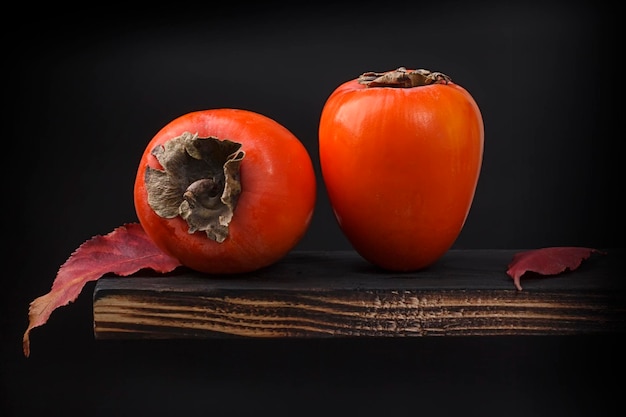The photograph showcases two vibrant orange persimmon fruits on a rustic wooden shelf against a stark black background. One persimmon lies on its side, revealing its lush green calyx, while the other stands upright, proudly displaying its perfectly round shape. Surrounding the fruits, delicate dark reddish-brown leaves are thoughtfully scattered to the left and right, adding a rich texture and contrast to the composition. The deep, almost fiery orange of the persimmons is accentuated by the interplay of the dark leaves and the natural wood grain, creating a visually striking and harmonious image.